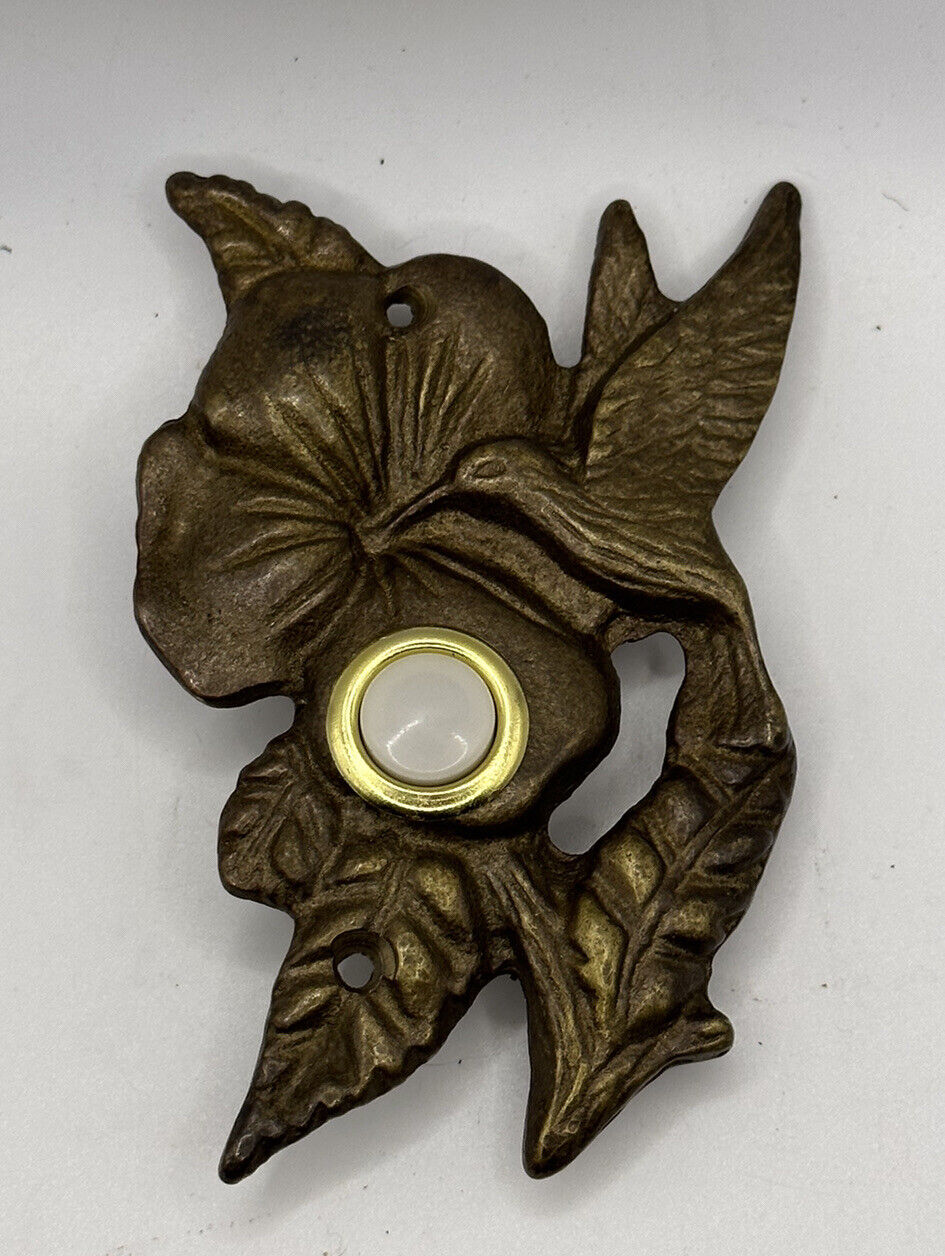The image depicts a detailed bronze doorbell cover designed in a floral and nature motif. The ornament features a hummingbird resting against a flower, likely a hibiscus, with intricate detailing including one smaller leaf sprouting from the top and two larger leaves at the base. This decorative piece, which could be mounted on a wall or placed on a table, measures approximately 10 to 12 inches tall and showcases a dark brown bronze color. At the center of the flower is a functional doorbell button, composed of a white button encircled by a gold ring, around four inches wide. Additionally, there are two strategic holes in the piece, one at the top of the flower and another at the bottom of the lower leaf, likely intended for screws to secure it in place.